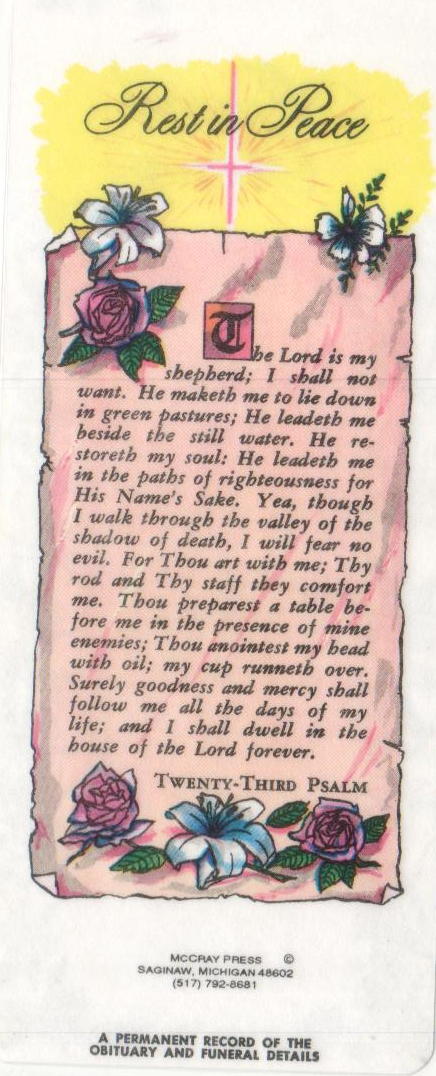This image is a detailed depiction of a funeral obituary card, resembling a bookmark and presented in a vertical rectangle form. At the top, it is inscribed with the phrase "Rest in Peace" in black, set against a yellow background. Below this, a pink cross with rays emanating from its center is prominently displayed. The main section consists of a pink rectangle framed by intricately drawn borders featuring an arrangement of red and white flowers with accompanying green leaves. Within this rectangle is an extensive section of text, which includes the 23rd Psalm: "The Lord is my shepherd, I shall not want. He maketh me lie down in green pastures…" and so forth, conveying a sense of serenity and spiritual reflection. At the bottom of the pink rectangle, additional text provides contact information and further details about the funeral. Beneath this section, on a white background, there are three more lines of black text, followed by two lines at the very bottom, which indicate this is a permanent record of the obituary and funeral details. The color palette includes white, yellow, black, pink, red, and blue, contributing to the solemn yet soothing aesthetic appropriate for a condolence card.